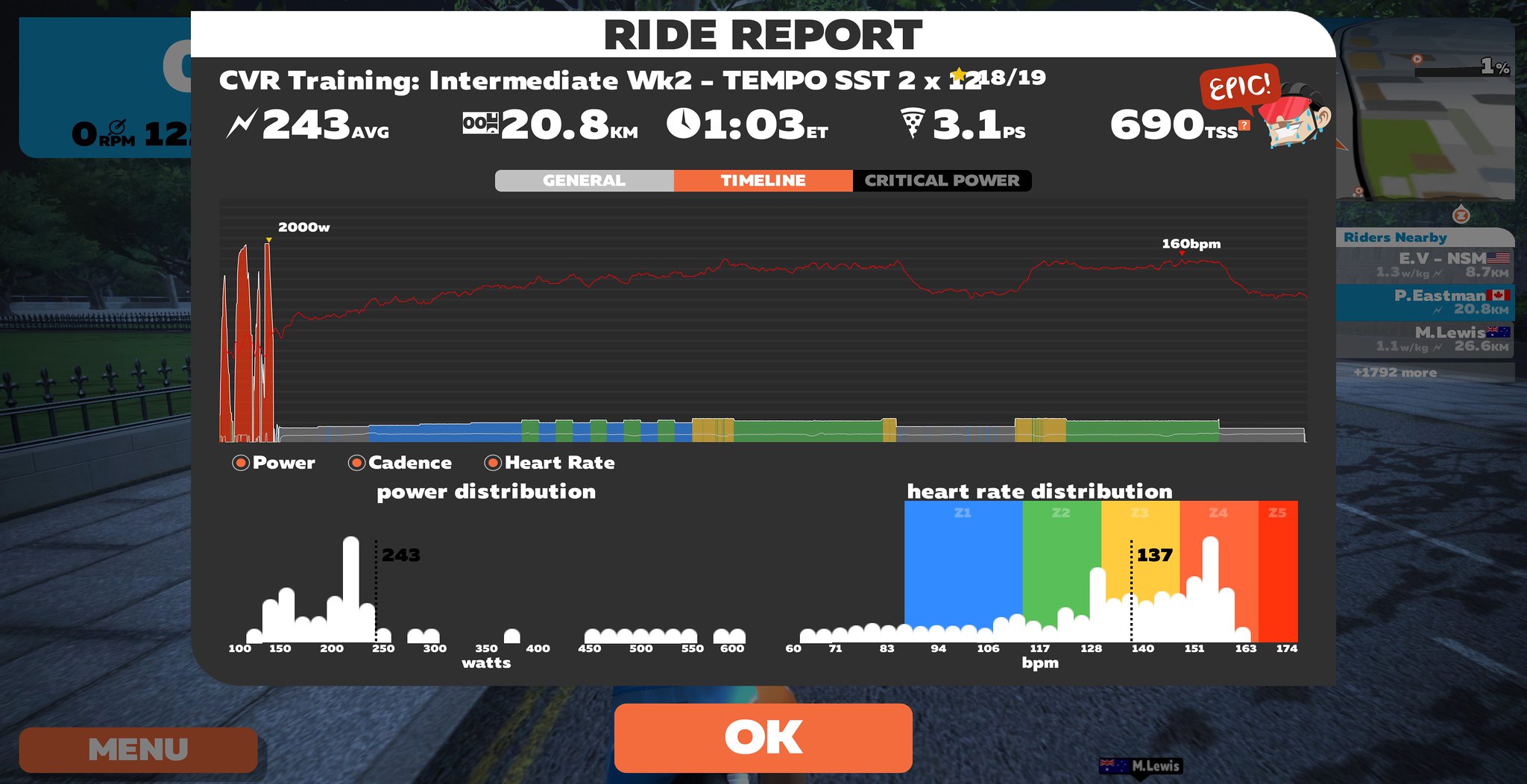This image is a detailed screenshot of an exercise dashboard, specifically a "Ride Report" from a computer application, likely related to cycling training or a virtual cycling game. At the top, the title "Ride Report" is prominently displayed. The session details immediately follow, indicating it's "CVR Training Intermediate WK2 - Tempo SST2 times 12, 18 out of 19." Key metrics are prominently featured below this title, including an average power of 243 Watts (represented by a lightning bolt icon), a distance covered of 20.8 kilometers (KM), a time of 1 minute and 3 seconds (shown with a clock icon), and a Performance Score (PS) of 3.1 (displayed with a slice of pizza icon), along with a Training Stress Score (TSS) of 690.

On the left side of the panel, a nearly solid red bar graph indicates heart rate distribution, suggesting intense activity, with a spectrum of heart rate zones in blue, green, yellow, orange, and red. At the bottom of the report, there's an orange "OK" button that can be clicked to close the window. Additional contextual details from the far left indicate labels for "Menu," while metrics such as power, cadence, and heart rate are specified, with watts and beats per minute also displayed. The dashboard presents a comprehensive overview of the workout session, with a layered window setup hinting at additional relevant information in the background.